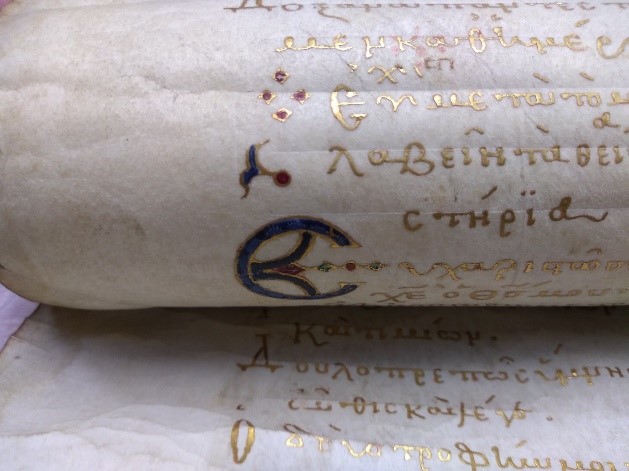The image is a close-up, color photograph of an ancient-looking scroll made from a whitish, tannish, possibly cotton paper. The scroll is partially unrolled, revealing paper edges that are slightly burnt and scorched. The paper has light creases throughout, adding to its aged appearance. The writing on the scroll is in a foreign language, possibly Arabic or another script, and is rendered in a metallic gold print that appears raised, giving it a textured look. Scattered across the scroll are small red dots and a prominent symbol resembling a navy blue 'C' shape outlined in gold, adorned with a flourishing, wavy, scalloped design inside. The 'C' shape also features stones in green and burgundy hues. The scroll rests on a light white sheet, providing a neutral backdrop that focuses attention on its intricate details and ancient script.